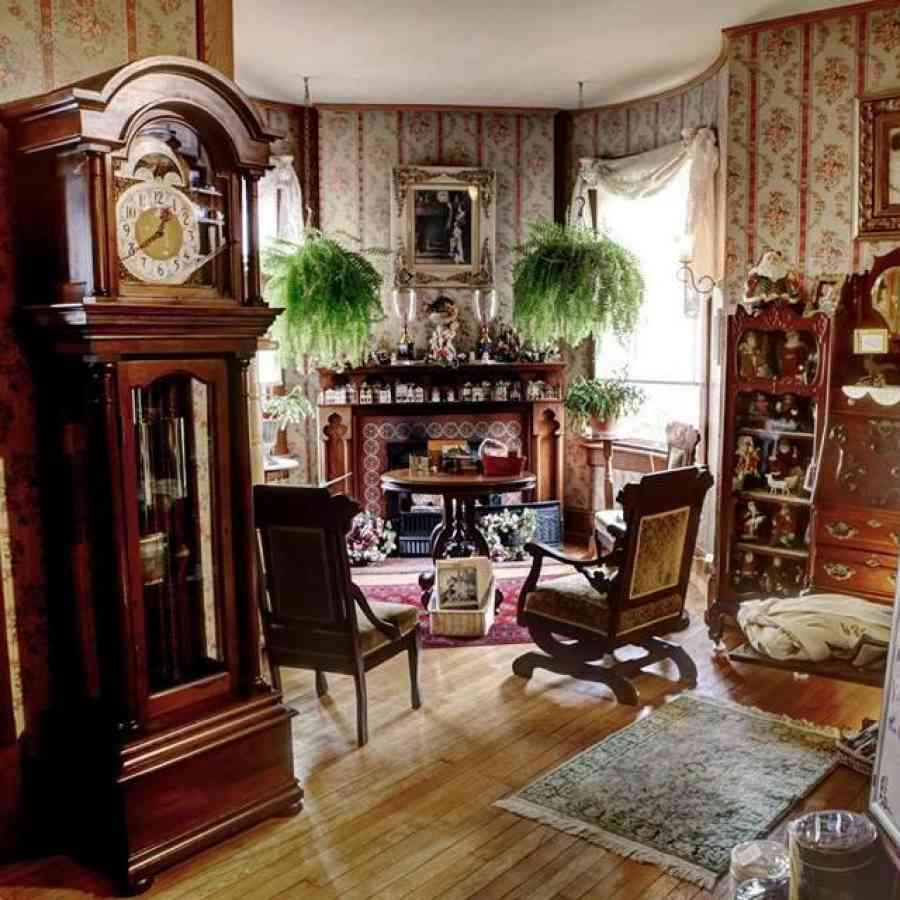The image depicts a Victorian-style room adorned in rich, dark brown mahogany tones. A prominent grandfather clock stands as a focal point, accompanied by a classic dark brown rocking chair with floral cushions. Next to it, there is another chair with a similar floral cushion, enhancing the room's vintage charm. The walls are covered in a floral-patterned wallpaper, which adds to the room's old-fashioned ambiance. Hanging plants, primarily ferns, contribute a touch of nature and greenery.

A dark wood mahogany cabinet lines one of the walls, showcasing an array of knickknacks and dolls. In a corner stands a fireplace, also crafted from mahogany, with a rug laid out before it. Atop a table nearby sits a basket filled with various items. Above the fireplace hangs a framed picture with a flowery border. The floor is light brown hardwood, partially covered by a small area rug positioned behind the chairs, tying together the room's cozy, antique aesthetic.